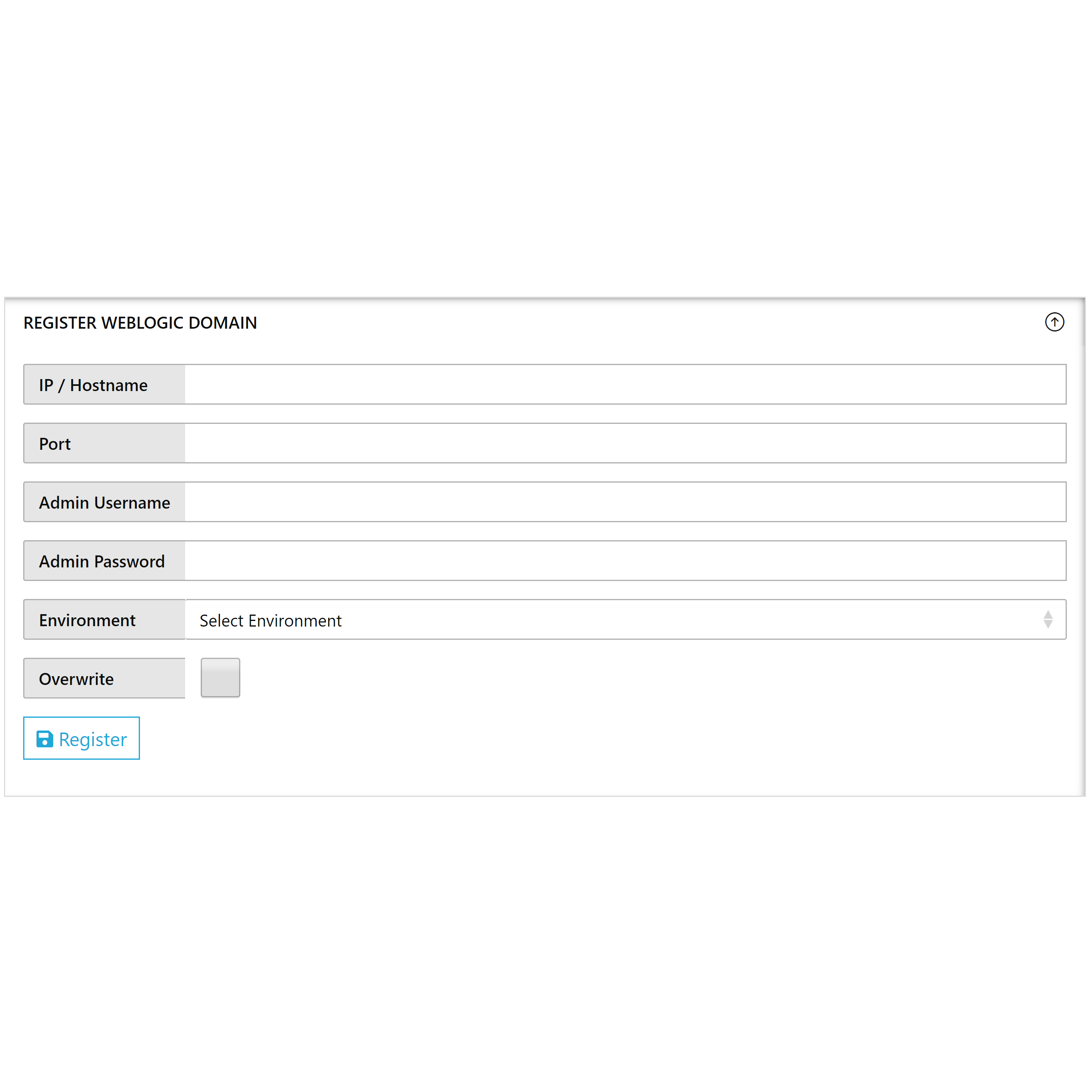The image displays a simple text entry screen titled "REGISTER WEB LOGIC DOMAIN" in all capital letters at the top. Below the title, the screen features a series of options with adjacent empty text fields, labeled as follows: IP Hostname, Port, Admin Username, and Admin Password. Each of these text fields is completely blank. 

The fifth option, Environment, is represented by a drop-down menu with the placeholder text "Select Environment," though the dropdown is not expanded, so the available environment options are not visible. 

The final option, Overwrite, is a checkbox that is currently unchecked. Unlike the previous fields, this is not a text entry field.

At the bottom of the screen, there is a blue icon button labeled "Register," which stands out against the rest of the screen's gray-toned elements. The interface is minimalist, featuring no other graphical or textual elements.